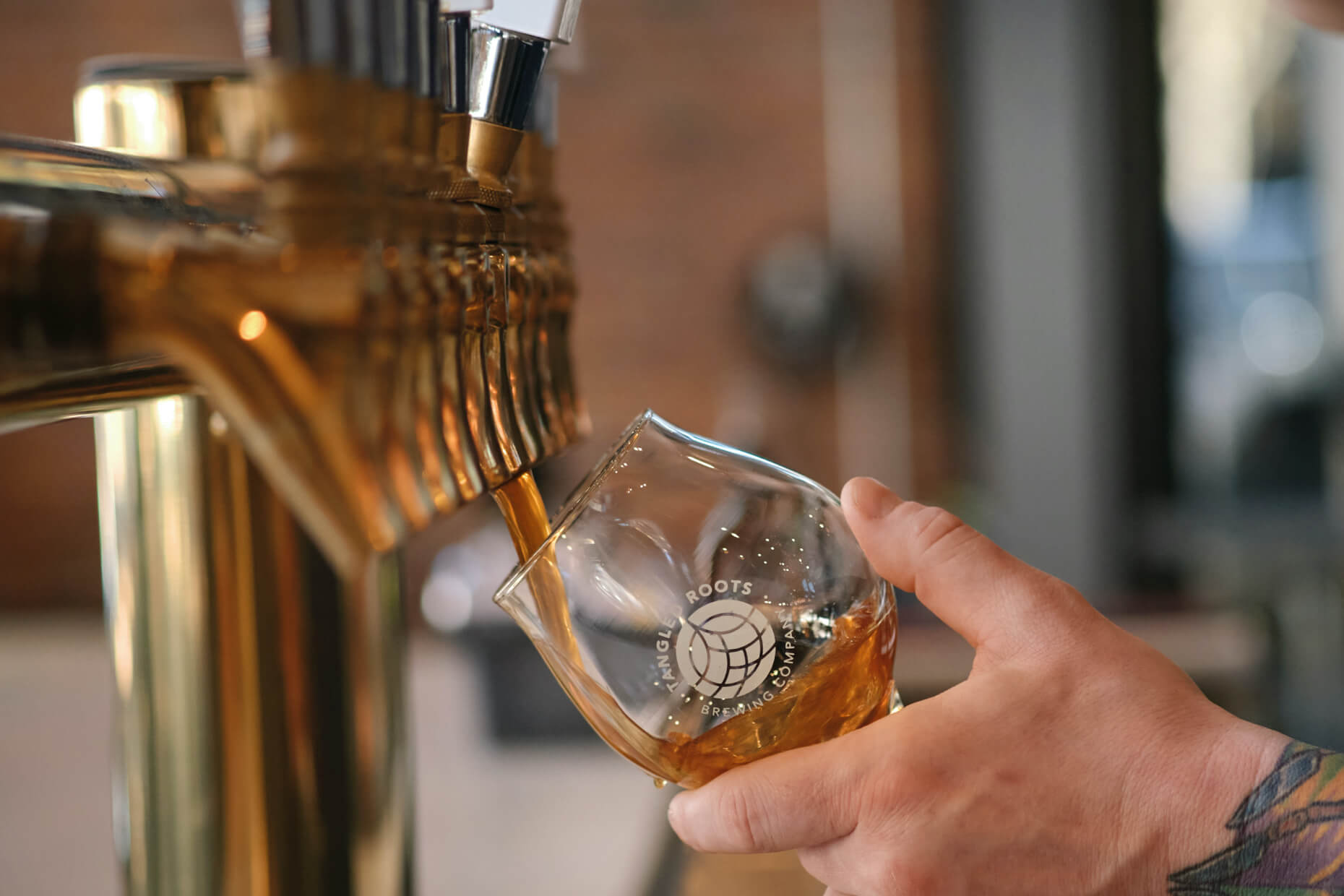The rectangular photograph captures a vibrant scene at a brewery or bar. In the center of the image, a round, transparent drinking glass adorned with a white logo that reads "Tangled Roots Brewing Company" is being filled with an amber-like beer. The glass is tilted to its side, gripped by someone’s left hand. Only the hand is visible, showcasing a colorful blue, purple, and yellow tattoo on the forearm. To the left, a brass beer tap with multiple spouts and black levers is prominently featured. The background, slightly out of focus, suggests a commercial setting akin to a brewery or restaurant, with a blurred brown-gray interior adding depth to the scene.